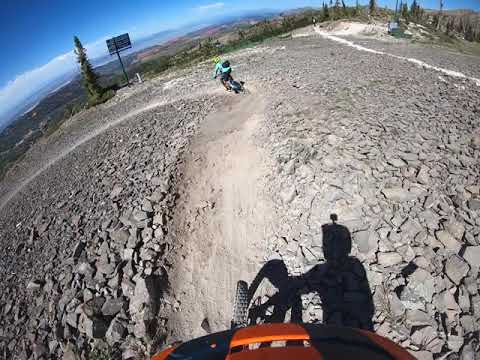This photograph, likely captured from a GoPro attached to a cyclist's helmet, reveals a dynamic scene of off-road biking. The image, slightly wider than it is tall, showcases a rugged dirt trail lined with rocks and mud. The trail starts at the bottom center, curving left as it recedes into the background. In the foreground, the orange frame and front wheel of the cyclist's bike are visible, along with the shadowy silhouette of the cyclist, indicating a camera mounted atop their helmet. Ahead on the rocky path, another cyclist in a green shirt and black shorts can be seen, possibly wearing a backpack. The background boasts a partially cloudy blue sky, with trees dotting the upper right and left quadrants. The landscape also features low hills and valleys, adding depth to the scene. This picturesque yet challenging biking route is vividly brought to life through the fisheye lens effect, accentuating the trail's curves and the terrain's intricacies.